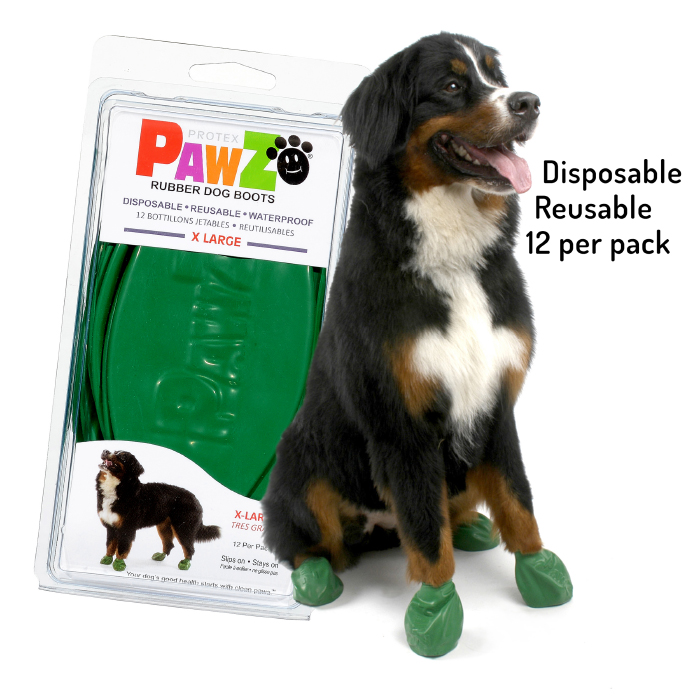The image features a sleek advertisement for a pet product against a pristine white background. Central to the composition is a large black dog with distinctive markings: a white belly, brown highlights around the eyes and legs, and additional white around the eyes. The dog appears to be slightly uncomfortable, wearing green plastic wraps on all its paws—both front and back. 

To the left of the dog is a clear clamshell container, displayed vertically and almost matching the dog's size. The container reveals green dog boots inside and bears a detailed label. The label prominently reads "Protex Paws Rubber Dog Boots Disposable, Reusable, Waterproof, 12," with additional text in another language. A photo of the same black, white, and brown dog sporting the boots is visible on the label along with the size description, "Extra Large." 

On the right, near the dog's mouth, the label reiterates in black letters: "Disposable, Reusable, 12 per pack." The dog, sitting upright on its haunches and looking off to the right, is the embodiment of the product's advertised utility and appeal.